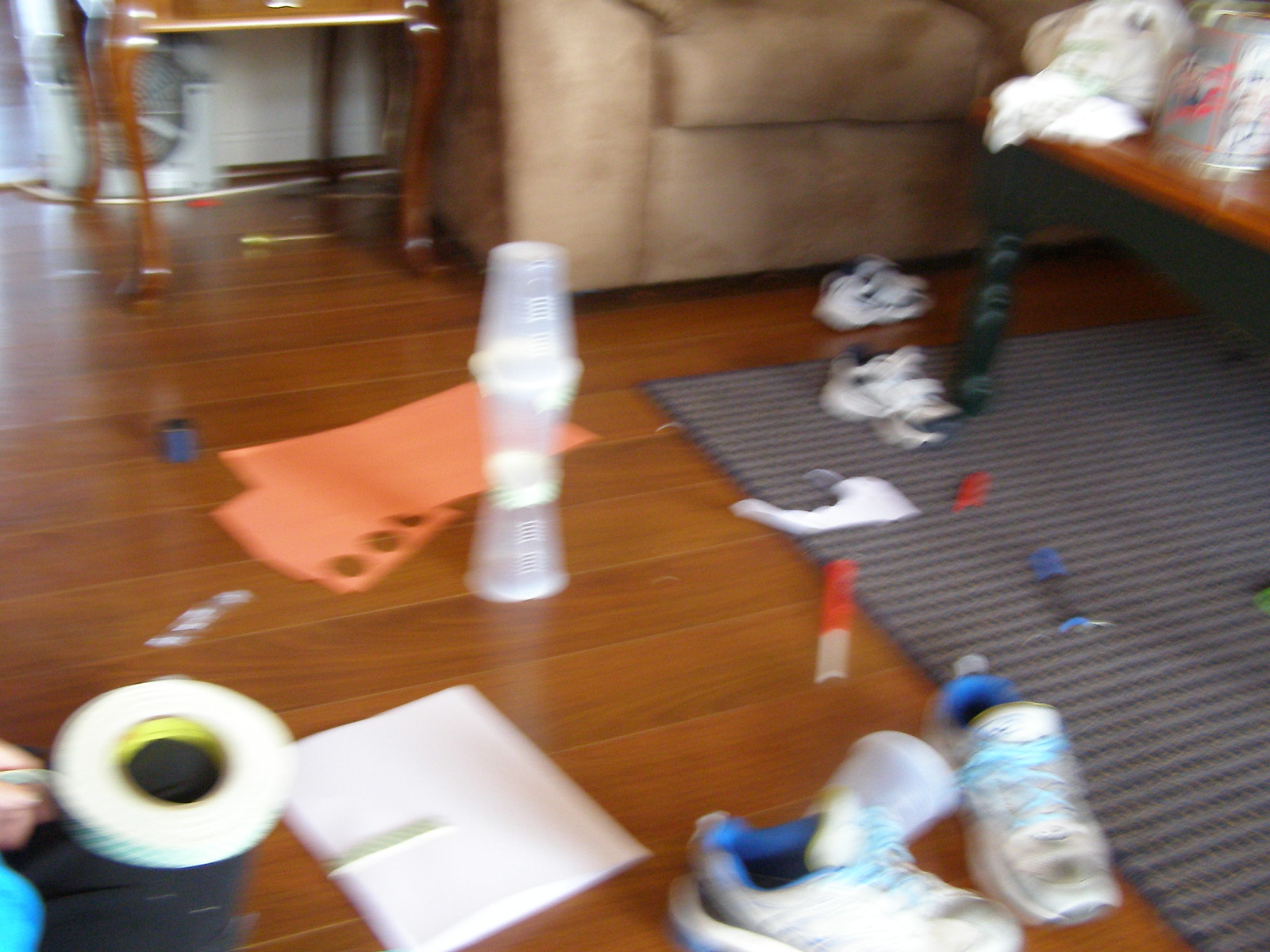The photograph captures a downward view of a cluttered living room floor, giving an impression of ongoing arts and crafts activities. The scene is set against a light brown, hardwood floor. In the upper portion of the image, the legs and underside of a brown wooden end table are visible. To the right of the end table, the bottom half of a light brown couch can be seen, showcasing the lower cushions. 

In front of the couch and towards the right side of the image, a blue and white rug is positioned. A light brown coffee table with a dark frame sits atop the rug, with visible plastic bags and miscellaneous items cluttering one of its corners. Near the visible leg of this coffee table, there's a pair of small white children's shoes, scattered pieces of paper, and pencils.

Moving towards the left center of the floor, another pair of white shoes with blue interiors can be observed. Close by, a white piece of paper lies off-center. Dominating the center of the image, a few cups are stacked on top of each other. There are also a couple of orange construction papers on the ground, one of which has three circles cut out of it. Finally, in the bottom left corner, a roll of tape rests on someone's knee, who is wearing black pants and is partially out of the frame.